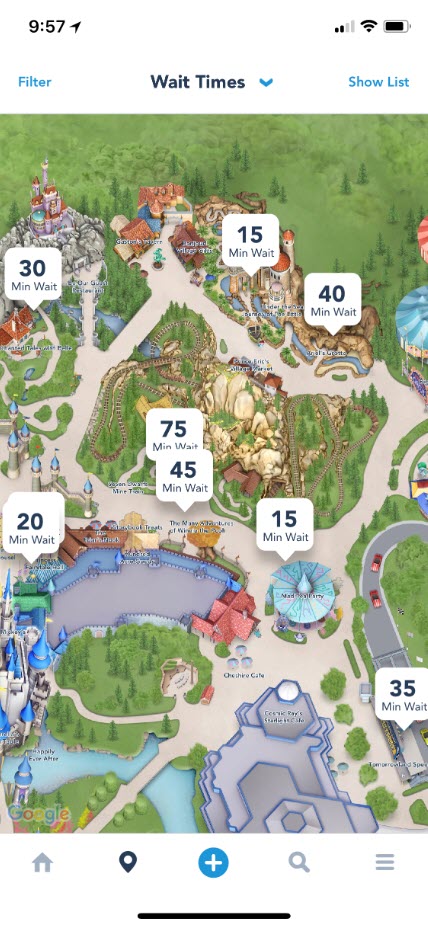The image in question depicts a colorful, illustrated map of an amusement park, viewed on a mobile phone screen. At the very top of the screen, the device displays the time as 9:57. To the right of the time, two solid bars indicate cellular signal strength, followed by the Wi-Fi icon and the battery icon. 

Beneath this status bar, on the left side, the word "Filter" appears in blue text. Adjacent to it, a blue drop-down box labeled "Wait Times" is present, accompanied by a down-pointing arrow. Further to the right, another white space separates the text "Filter" and the option "Show List" which is also in blue.

The map itself is richly detailed with various green areas representing different sections of the park. Overlaid on this map are small rectangular or square boxes, each containing a wait time and marked with a small triangle pointing to the respective ride or location.

Specifically, the wait times are distributed as follows:
- Top left corner shows a ride with a 30-minute wait.
- Below that, another ride indicates a 20-minute wait.
- In the center of the map, there are wait times of 75 minutes and 45 minutes for two different attractions.
- Slightly to the right of the center, a ride shows a 15-minute wait.
- Further to the right, another attraction has a 40-minute wait.
- Moving downward from these points, a box indicates another 15-minute wait.
- Finally, at the bottom right corner, there is a 35-minute wait displayed.

Additionally, the map includes illustrations of the different rides located at the park, visually tied to their respective wait times.